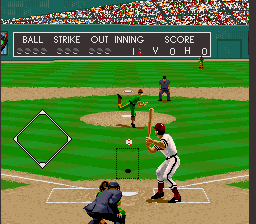This small, square, pixelated screenshot captures vintage baseball video game action from a behind-the-plate view. In the foreground, the umpire is bent over behind the squatting catcher, while the batter stands poised with his bat raised behind his head, ready to swing at the incoming ball. The pitch, depicted as a black dot, is on its way toward the batter, with its anticipated position indicated by a black box over home plate. The pitcher, dressed in a green uniform with his leg cocked high behind him, has just released the ball. A white triangle icon to the left displays the empty bases against a backdrop of the diamond, and another umpire can be seen near the shortstop area.

In the distance behind the pitcher, the second baseman and a cheering crowd fill the background. The top of the screen features a banner displaying "ball," "strike," "out," "inning," and "score," with dots beneath the categories yet to be illuminated. The game is in the first inning, as indicated by the scoreboard showing "V 0 H 0," signifying no runs scored by either team so far.